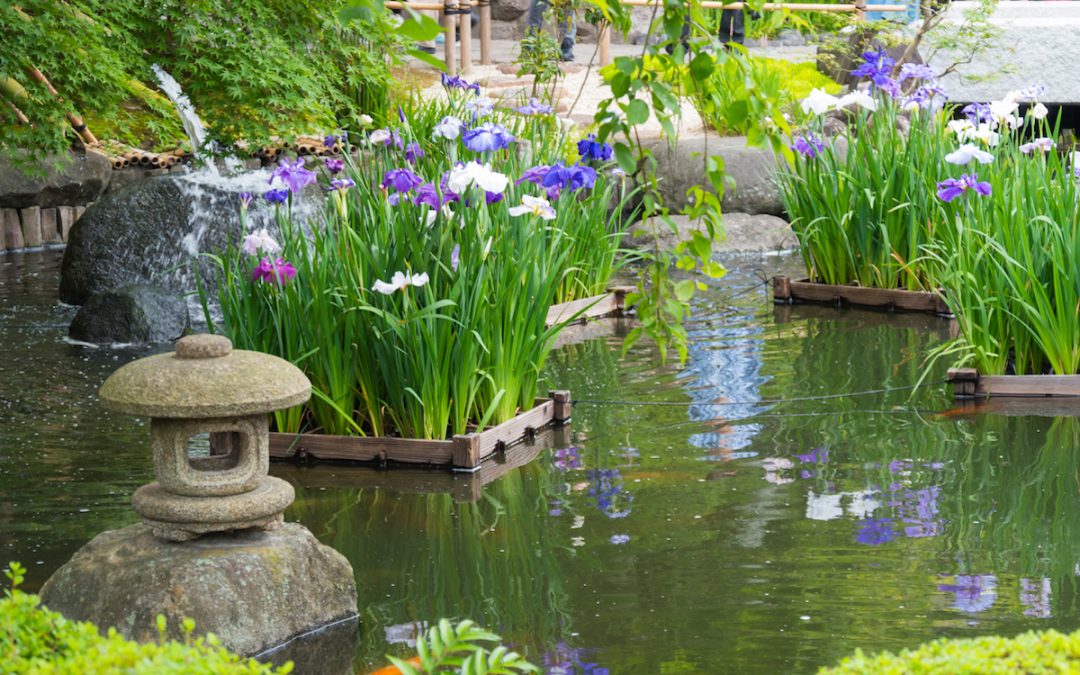This is an outdoor photograph taken of a serene Japanese garden pond featuring a man-made, Asian-style design. Central to the pond are four wooden platform planters, brimming with vibrant flowers on tall green stems, predominantly showcasing shades of pink, white, purple, and blue-violet. The platforms are interlinked with wire cables, giving the appearance of floating gardens. 

In the background, a picturesque arrangement of dark brown and gray rocks is visible, further emphasizing the natural aesthetic of the scene. Bamboo shoots emerge from the side of a hill, creating a cascading water feature that flows into the pond. Adding to the traditional ambiance, the foreground features a stone structure resembling a carved lantern, indicative of typical Japanese architectural symbolism.

A temple-like structure with distinct Asian design elements can also be seen in the foreground, with a garden pathway or stone area for walking extending into the background. Sparse vegetation and a somewhat overcast sky suggest a tranquil and contemplative atmosphere in the image.